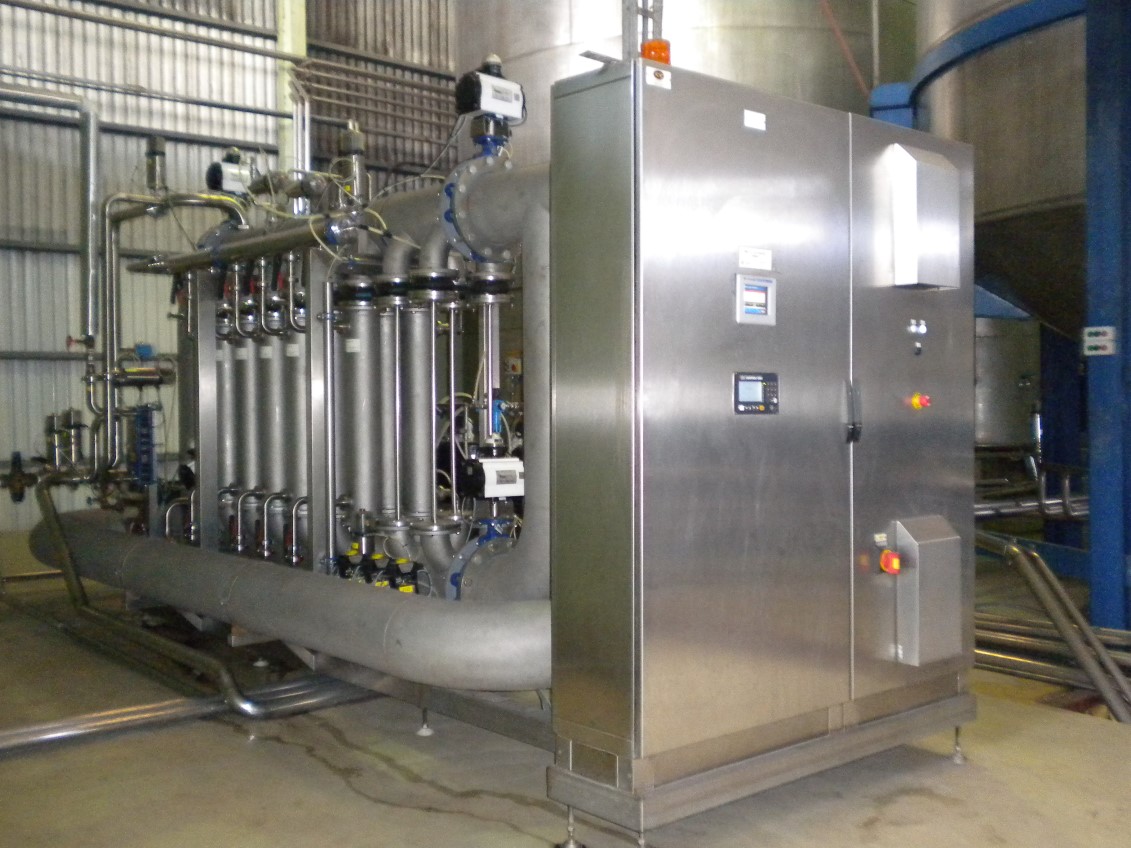The image depicts a large, well-maintained water treatment machine standing on skinny legs with suction cup ends, placed on a cement floor with visible water stains. The machine resembles a two-door refrigerator with stainless steel or chrome-colored front doors equipped with two small handles in the middle. The front of the machine features various control elements, including a keypad for code input, reflective lights, and some venting. On the left side, there are light-reading panels. The back is densely packed with long, vertical tubes, both metal and plastic, in colors such as blue, white, and yellow, along with many wires on the top. The entire setup is situated in a metal warehouse or basement environment, highlighting its commercial application.